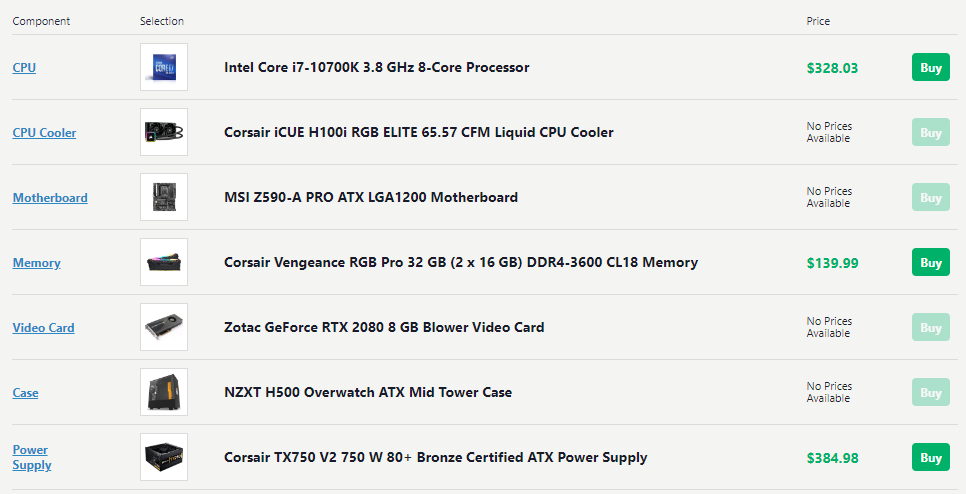The image depicts a generic website designed for selling computer components, lacking any identifying marks to indicate its exact source. The interface is divided into four main columns of information.

The first column on the left lists the categories of computer components available for purchase, including CPUs, CPU coolers, motherboards, memory, and video cards.

The second and largest column features a small thumbnail image for each product, accompanied by a detailed description. For instance, one entry showcases a small Intel logo alongside the text "Intel Core i7," indicating it is an Intel Core i7 processor.

The third column displays the price of each component in U.S. dollars, with the prices listed in green font. Some entries may show "price not available" if the cost is not listed.

The fourth and final column contains a green button for each item, which shoppers can click to add the product to their cart if they wish to make a purchase.